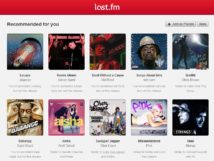The image is quite blurry, and a red box at the top reads "LCST.FM." Below this red box, the text "Recommended for you" is displayed. Various album covers are featured, including:

1. An album that appears to show someone inside a clear capsule.
2. Another cover with a man who resembles Billy the Kid, smoking a cigar and wearing a distinctive hat; the background is blue and his hat is gold with a black brim.
3. A cover displaying just the silhouette of a man's face against a black background.
4. An album cover with stylized text that could be "PIDE" in pink letters, featuring a woman with blonde hair streaked with pink at the top. She is laying down, wearing a white top.
5. A cover showcasing a girl named Christy, dressed in a blue denim long coat, a blue crop top, and a rust-colored skirt.
6. An album titled "Asewa" or "Asa," featuring a pink background, though the background details are unclear.
7. A cover with a man whose face is styled like Frankenstein's monster; he is making an "O" shape with his fingers next to his eyes, and the text includes the word "Alliance."

Overall, the image captures a selection of various eclectic and visually striking album covers, each with distinct and memorable features, recommended to the viewer.